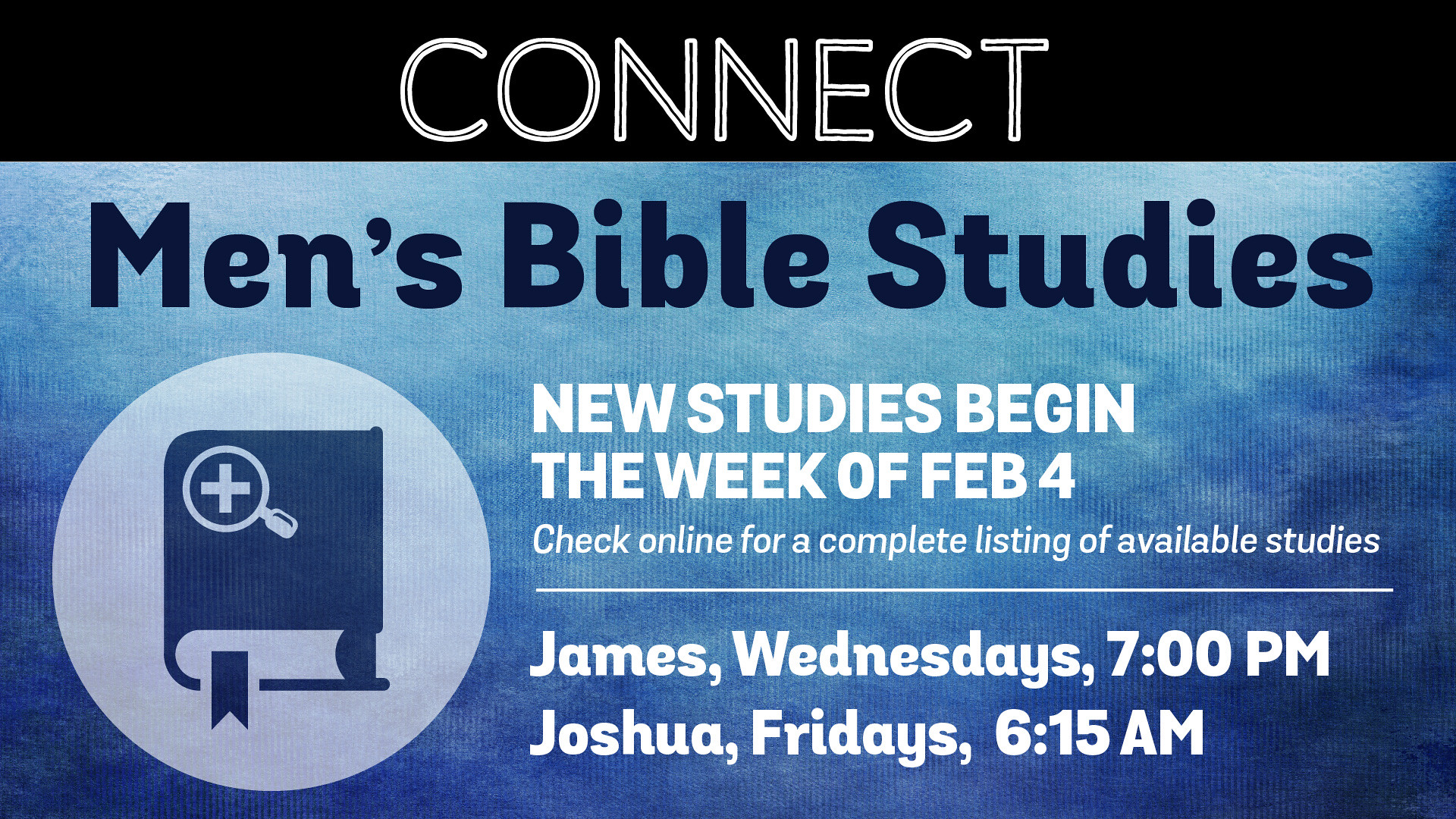This advertisement for men's Bible studies features a striking design with a bold, black stripe at the top displaying the word "CONNECT" in prominent white writing. Below this stripe, the background shifts to a mix of light and dark blue shades, reminiscent of a tie-dye effect or an underwater scene. Centered within this blue backdrop, "Men's Bible Studies" is written in dark navy font. Subsequent text in white font announces, "New studies begin the week of February 4. Check online for a complete listing of available studies." Specific study groups are highlighted next: "James - Wednesday 7 PM" and "Joshua - Friday 6:15 AM." To the left side of the text, there is a circle with a gray background, featuring a graphic of a blue hardcover Bible with a bookmark protruding from its pages. A plus sign or cross-like symbol appears on the upper left side of the Bible.